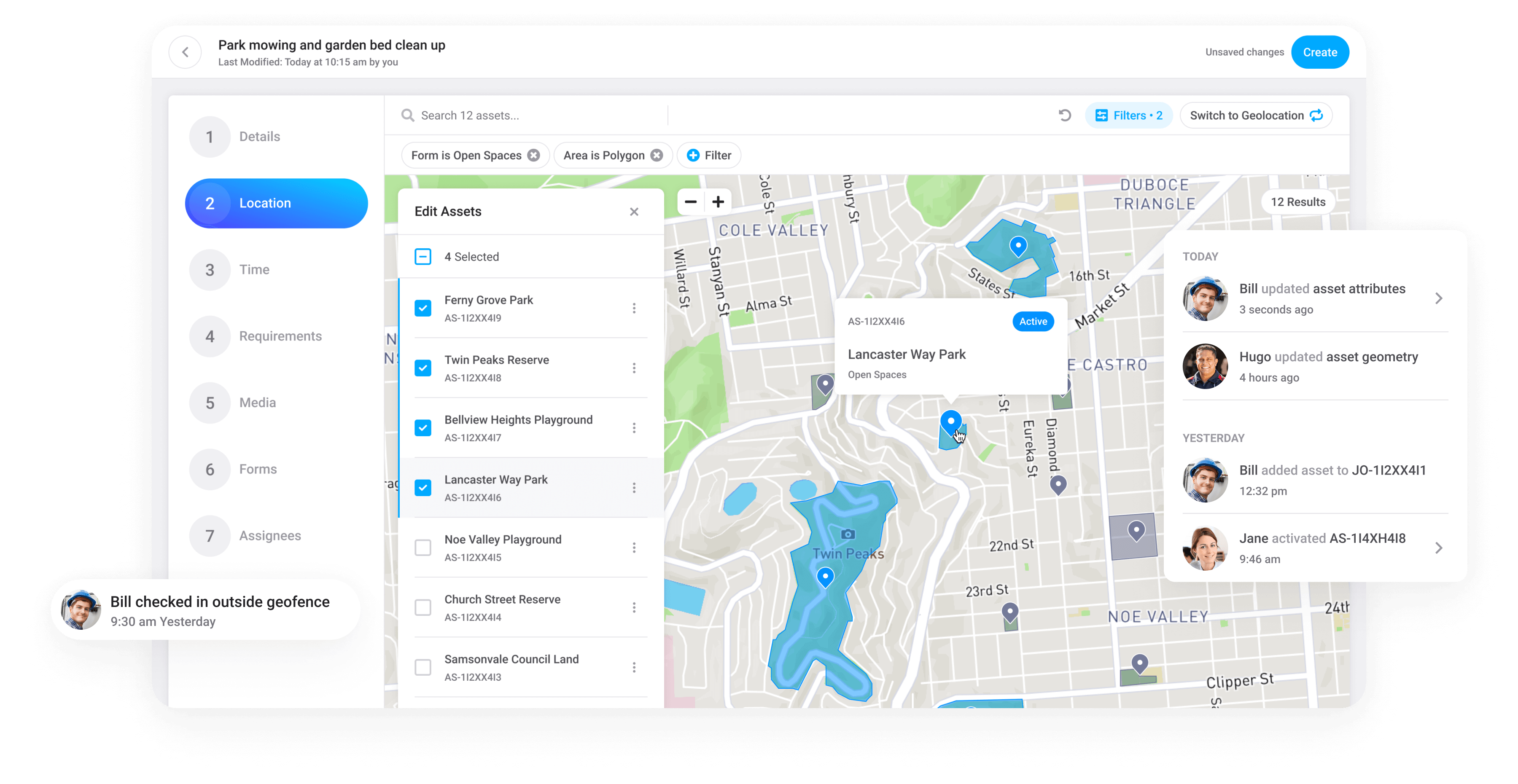This screenshot showcases a detailed task management interface for park maintenance activities. At the top, the task is titled "Park Mowing and Garden Bed Cleanup," with the field verification timestamp noted as "last verified today at 10:15 AM." To the top left, a back arrow is visible, allowing navigation to a previous screen, while on the top right, there's a "Create" button for initiating new tasks.

On the left-hand side of the interface, a vertical list numbered one through seven outlines different task components: Details, Location, Time Requirement, Media, Forms, Assignees, and more. Below this list, an entry notes that "Bill checked in outside geofence at 9:30 AM, Tuesday," along with options to "Edit your assets."

The main portion of the screenshot displays a map featuring various streets and landmarks, such as Clipper Street, Noe Valley, 23rd, 22nd, Diamond, Eubanks, Coal Valley, and Dupont Triangle. Points on the map appear to correspond with specific task locations.

The screenshot also includes a log of recent updates, indicating team activity: one person updated their contributions three seconds ago, another adjusted their geometry four hours ago, and additional activities from the previous day are listed as well.

This comprehensive visualization aids in tracking and managing park maintenance tasks effectively.